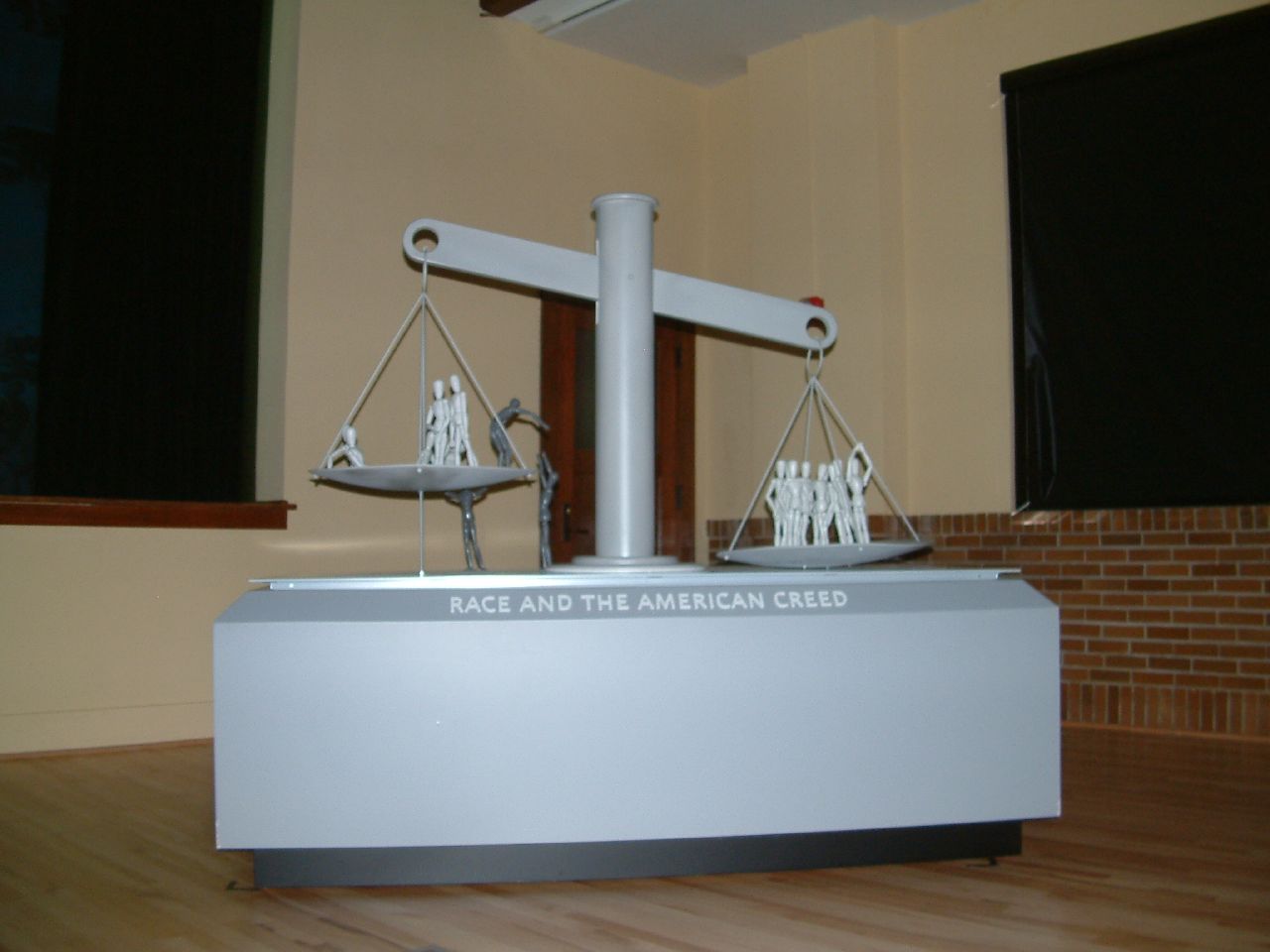The photograph, taken indoors, showcases a large, gray, metal art installation designed to resemble a justice scale, positioned in the center of a room. The impressive structure rests on a rectangular base inscribed with the phrase "Race and the American Creed" in lighter gray letters. The left scale, elevated higher, supports two white figures and one black figure struggling to climb. The lower right scale is heavily laden with numerous white figures. The setting includes beige walls with a salmon hue, a wooden floor, and a red brick section on the far right. Windows are covered with black tarps, obstructing any outside view. In the background, there's a red door and some black shades covering additional windows, adding to the room's unique atmosphere.